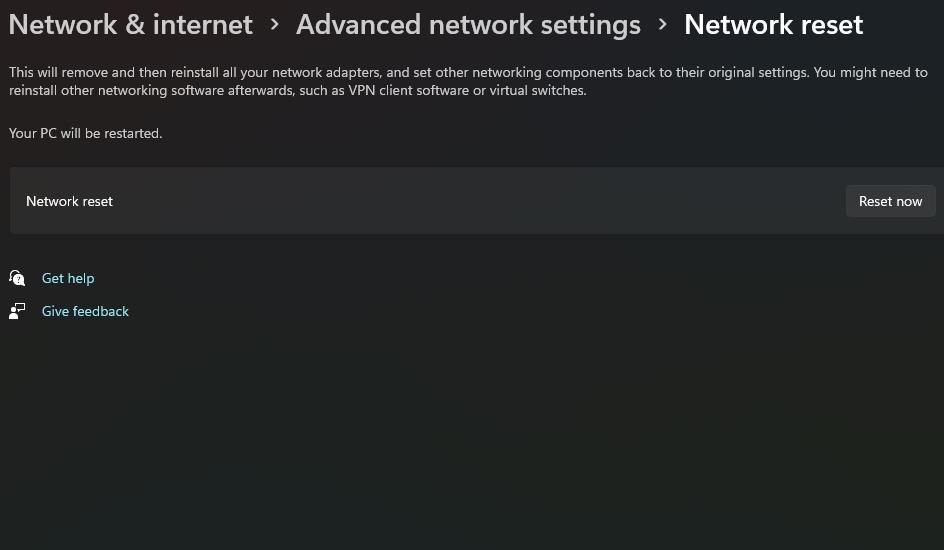A screenshot of the "Network Reset" settings within the "Advanced Network Settings" panel. The background is predominantly black. At the top left, in very large white letters, it reads "Network & Internet." To the right, an arrow points to "Advanced Network Settings," leading to another arrow pointing right, highlighting "Network Reset" in white.

Beneath this, a detailed explanation is provided in small white letters: "This will remove and then reinstall all your network adapters and set other networking components back to their original settings. You might need to reinstall other networking software afterwards such as VPN client software or virtual switches." 

On the left side, text in white reads, "Your PC will be restarted." Adjacent to this, a black box in the center displays "Network Reset" in white letters, while to the right, a black button with "Reset now" in white text is visible. 

Below, there is a chat bubble icon with "Get help" in blue font to its right, followed by a person icon with "Give feedback" in small blue letters to the right.